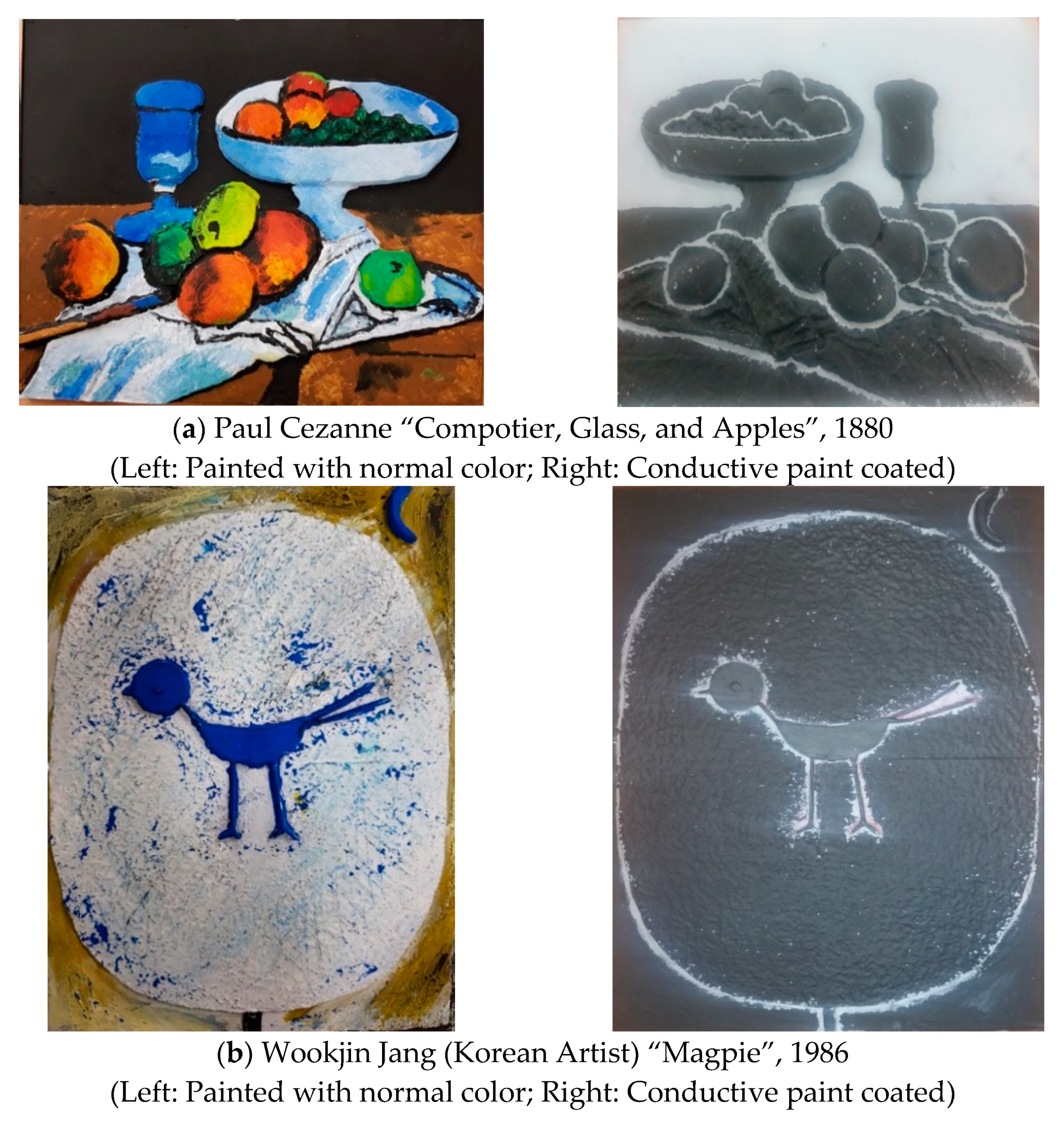This image depicts a textbook page that evaluates old paintings using both normal and conductive paint coatings. On the left side of the page, two artworks are displayed in their original colors. The top image features Paul Cézanne's "Compotier, Glass, and Apples" from 1880, depicting a simple yet detailed arrangement of a fruit bowl, scattered fruits, and a glass. Below it is Wook Ching Jang's "Magpie," a 1986 painting of a blue and white bird on two wide legs. The right side of the page offers an x-ray-like view of these paintings, showing them in dark gray and white due to a conductive paint coating. This method allows for the detection of any tampering with the original artwork by highlighting differences between the color painting and the conductive paint outline. Both paintings showcase the left side painted with normal colors and the right side with conductive paint, illustrating a study of artistic authenticity and preservation techniques.